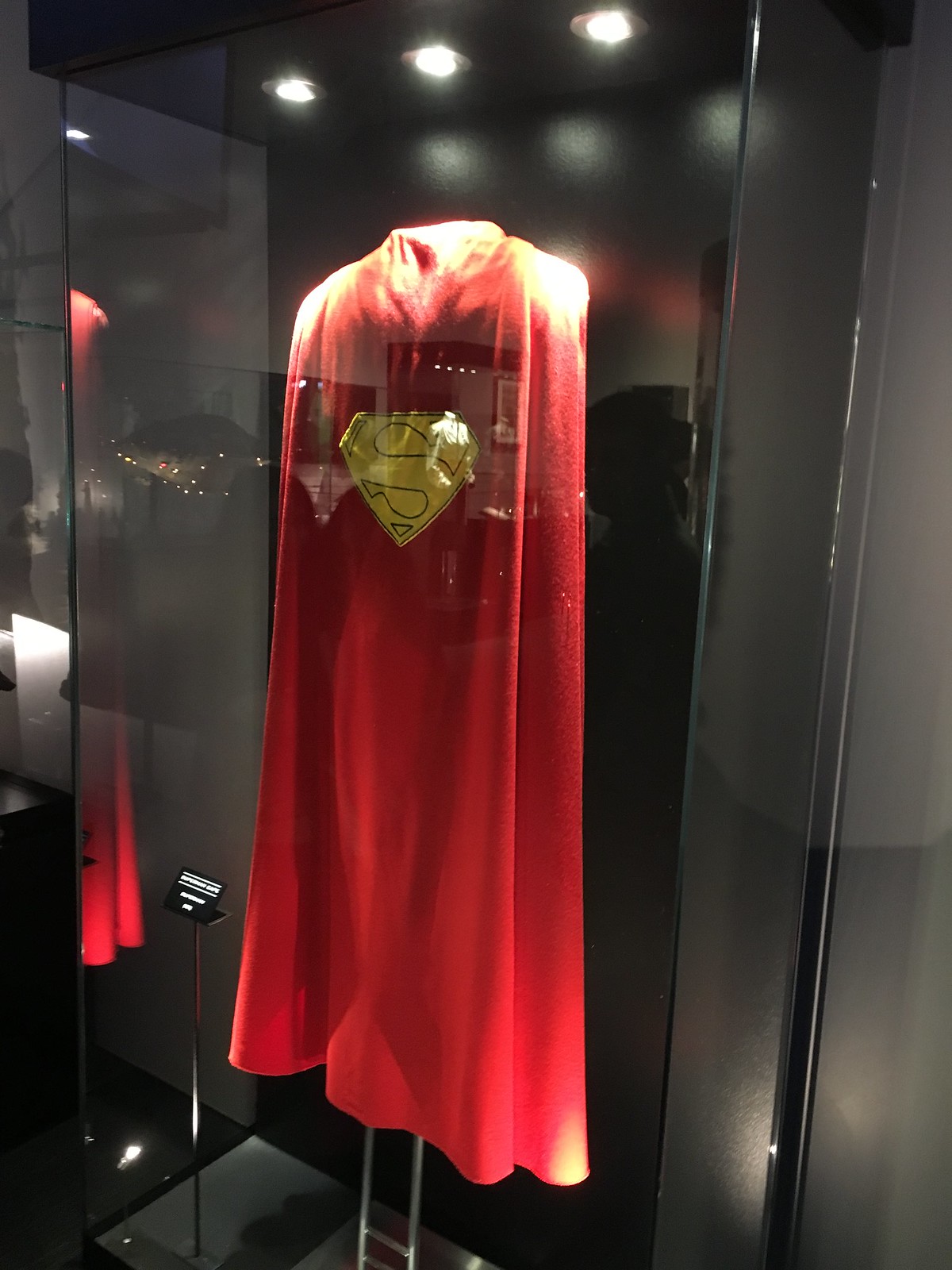This image depicts a red Superman cape displayed within a glass case, illuminated by three overhead can lights. The cape features a yellow Superman logo with a black outline both around the outer edge and the iconic 'S' in the center. Inside the case, a small black placard mounted on a black pole provides information, but the white text is too small to read at this resolution. Reflections on the glass case include an indistinct internal reflection of the cape and possible reflections of the person taking the photo. The backdrop includes a dark wall that enhances the display, and to the left, another exhibit partially obscured by what could be an umbrella or tarp can be seen. This setting suggests the photograph was taken at a museum or exhibit dedicated to Superman and comics. The display stand gives the impression that the cape is draped over invisible shoulders, further adding to its heroic presentation.